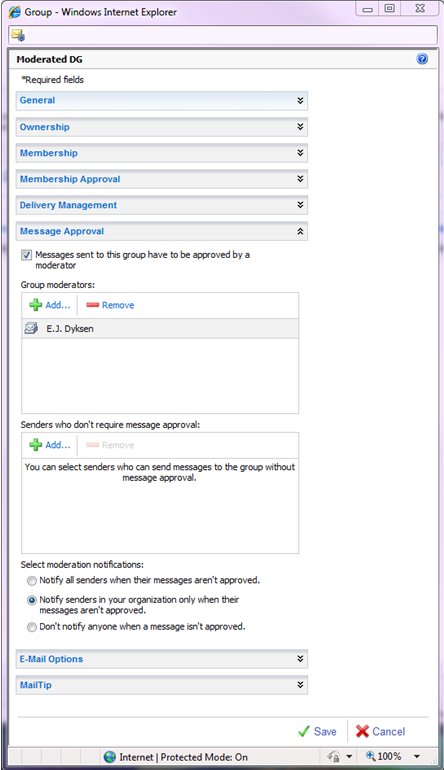This is a detailed screenshot of a settings menu within Windows Internet Explorer. At the top of the window, there's a blue title bar. On the left end of this bar, there's the Internet Explorer icon, represented by a blue 'E' with a slash through it. Next to the icon, in black font, it reads "group - Windows Internet Explorer." On the right side of the title bar, there are three standard window control buttons: a minus symbol (minimize), a square symbol (maximize/restore), and an X symbol (close).

Directly below the title bar is a white address bar with a folder icon on the left end. 

Below the address bar is the main settings interface. The first section is labeled "Moderated DG." Underneath this, there's a section labeled "Required Fields," marked by a small asterisk on the left.

Further down, there are several blue drop-down menus, each with darker blue font. The categories of these menus are as follows:
- General
- Ownership
- Membership
- Membership Approval
- Delivery Management
- Message Approval

A checkbox reads, "Messages sent to this group have to be approved by a moderator." Below this, there's a section labeled "Group moderators:" followed by an "Add" button (designated with a plus sign) and a "Remove" button (designated with a minus sign). The current group moderator listed is "E.J.Dykeson."